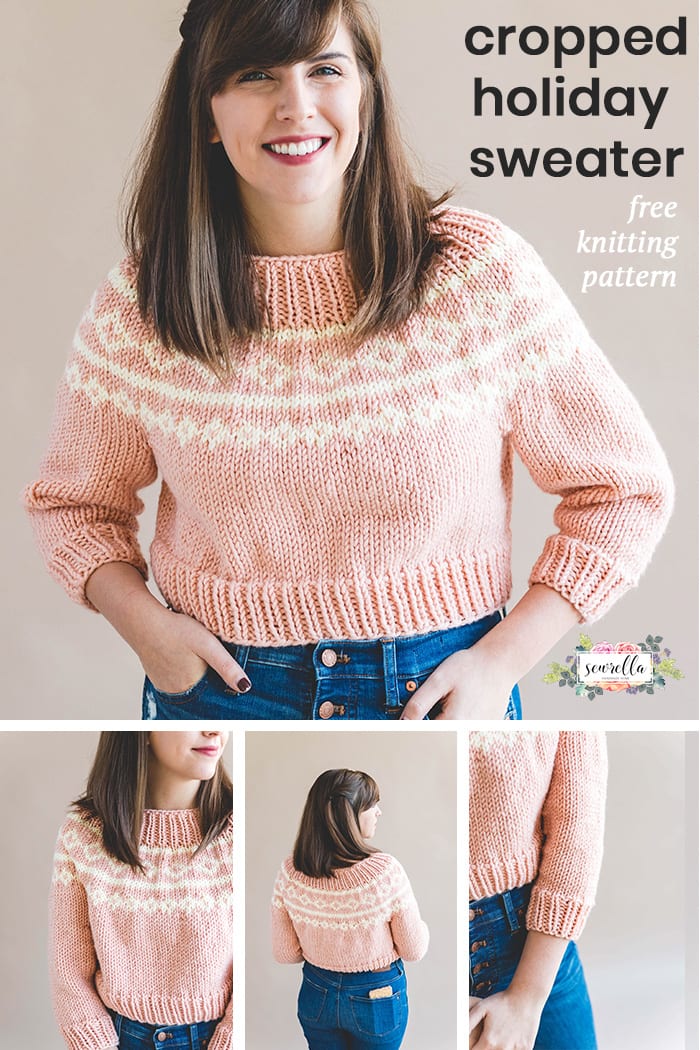The image appears to be an advertising collage from a magazine, promoting a knitting kit for creating a "Cropped Holiday Sweater." The main photograph showcases a woman with long brown hair, wearing a light pink sweater adorned with white stripes below the shoulder area, paired with light blue jeans. She stands against a light gray background, smiling warmly with her hands in her pockets. The top right corner of the image contains text that reads "Cropped Holiday Sweater, Free Knitting Pattern." Surrounding the main photograph, there are three smaller images providing different views of the sweater, depicting its front, back, and sleeves. The details highlight the well-designed and neatly decorated elements, including ribbed sleeves at the cuffs. In the bottom right corner, there is a logo surrounded by flowers with cursive text inside a white box, although the text is too small to be clearly read.